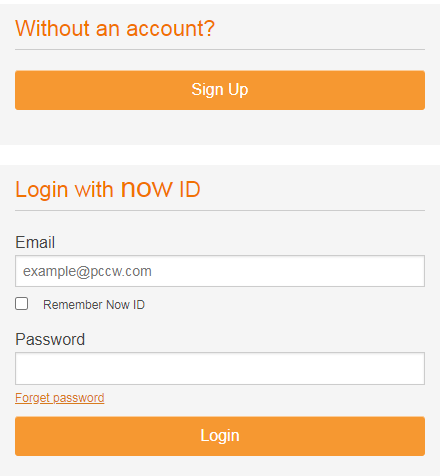The image showcases an account signup or login page with a gray background. At the top, bold orange text states, "Without an account." Below this, an orange "Signup" button invites new users to create an account. Further down, orange text that reads "Login with NowID" precedes a blank field labeled "Email," suggesting where users should input their email addresses. The placeholder text in this field is "example@pccw.com." Adjacent to this field is an unchecked checkbox labeled "Remember your NowID," which offers to autofill the email for future visits.

Underneath the email section, black text labels a blank field as "Password," with an orange "Forgot password?" link situated nearby. The page also features a prominent orange "Login" button with white text. The primary login interface, encompassing the input fields, is designed with contrasting white boxes against the gray background. The text throughout the image alternates between orange and black, indicating prompts and interactive elements. This page is clearly intended for users to either create a new account or log into an existing one.